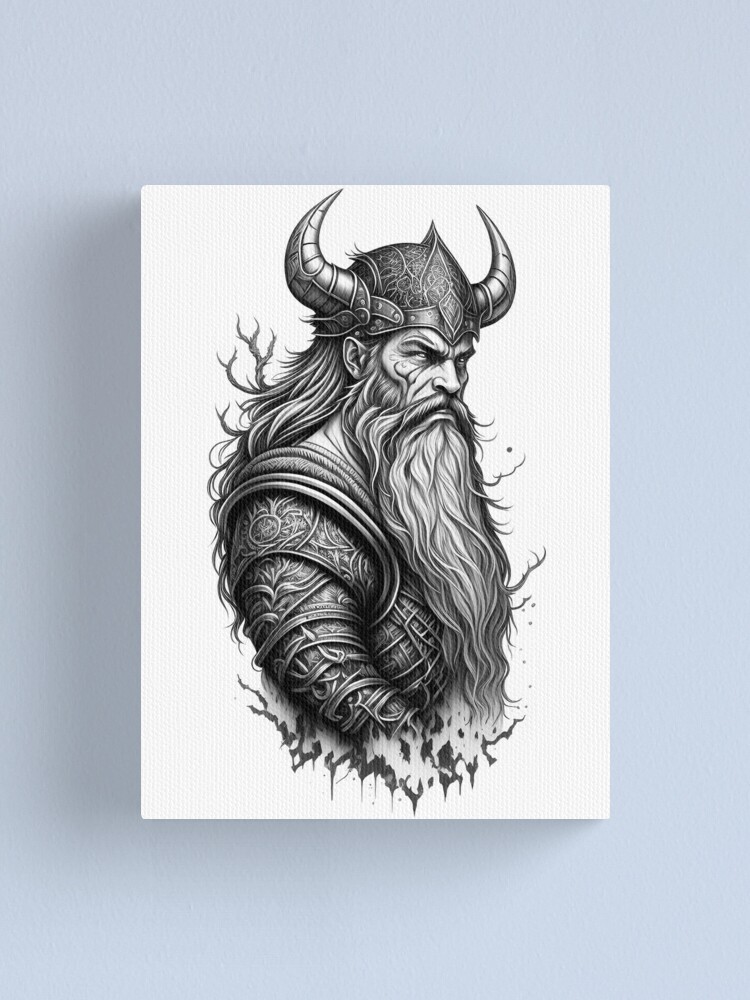The image is a detailed black and white sketch of a fantasy Viking character rendered on a piece of card with a light grayish-blue background, possibly created with charcoal or pencil. The Viking, facing to the right side of the frame, is depicted in a rugged, intense manner with an angry or determined expression. He sports a helmet adorned with two protruding horns and intricate, geometric, and organic designs. His armor, composed of numerous metal pieces, covers his upper torso to the waist, with no lower body parts visible. The Viking's long flowing hair, bushy beard, and prominent mustache enhance his fierce appearance, while his ears slightly protrude from behind his hair.